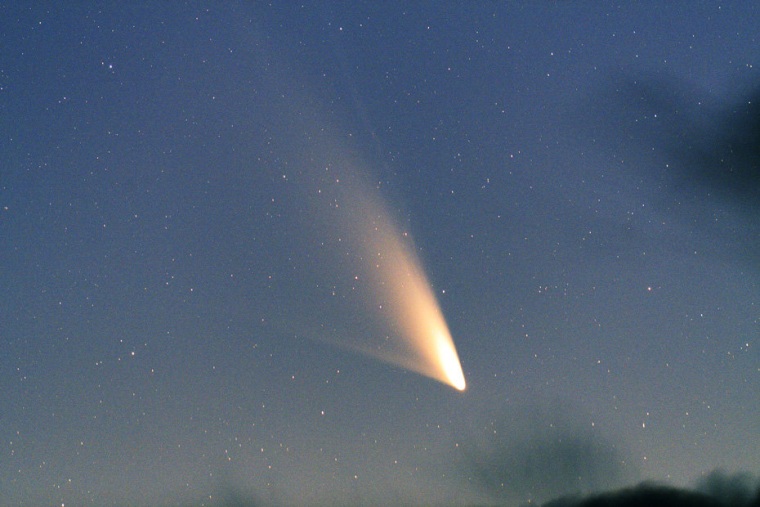In this photograph, taken in the early evening hours, a striking celestial event unfolds in the night sky. Against a backdrop of deep blues that gradually lighten toward the bottom, countless white stars punctuate the expansive heavens. Positioned near the lower center and slightly to the right, a brilliant comet or asteroid hurtles towards Earth, its head a dazzling white with a bright yellow core. This heavenly body leaves behind a long, luminous tail that fades into a deep yellow and slightly reddish hue as it stretches almost to the top of the image, becoming hazier and more diffuse. Dark clouds or gas formations frame the sky in the bottom right and top right corners, adding to the vibrant contrast. Just above the horizon, a faint sliver of Earth is visible, grounding the dramatic celestial display in the terrestrial realm. This vivid scene captures the awe-inspiring beauty of a comet or asteroid streaking through the twilight sky.